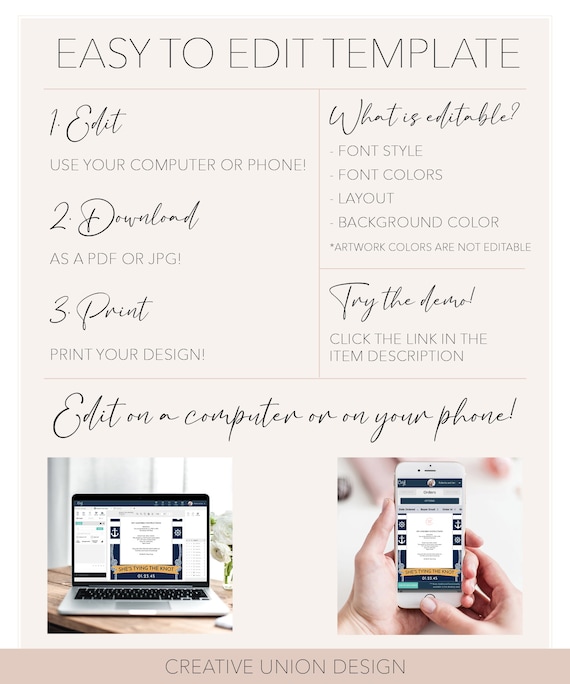The image appears to be an informative poster or infographic with an ecru, beige-ish background. At the top, it prominently displays the title "Easy to Edit Template." The poster is divided into several boxed sections, demarcated by darker beige lines. 

The first section contains a step-by-step guide on how to use the template:
1. **Edit:** Utilize your computer or phone.
2. **Download:** Save your design as a PDF or JPEG.
3. **Print:** Print your custom design.

The second section outlines editable elements:
- Font styles
- Font colors
- Layout
- Background color

It includes a note stating that "artwork colors are not editable."

The third section invites users to "Try the Demo" by clicking the link provided in the item description.

In the bottom third of the page, there's a message that says "edit on a computer or on your phone," accompanied by images of a Mac computer and an older model iPhone, both displaying web pages. At the very bottom, on a solid darker beige bar, it reads "Create a Union Design".

The overall layout is user-friendly and visually guides the viewer through the process of customizing a template using a computer or mobile device.